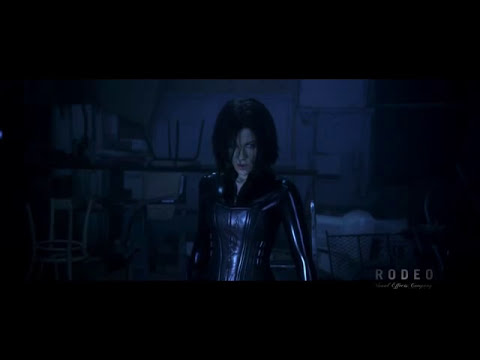The image appears to be a dark, underexposed screenshot from a video game or a TV/computer screen, framed with a black border. Central to the scene is a woman with long, dark hair, dressed in a black, skin-tight bodysuit that appears to be made of leather or latex. The setting behind her suggests she is in an industrial room, like a warehouse, with visible elements such as stacked tables to the left and a possible chair to the right. The scene is dimly lit, predominantly by a light that could be white or blue, possibly suggesting moonlight. The woman's expression conveys anger or determination. In the lower right-hand corner of the image, the word “Rodeo” is visible in white text, accompanied by smaller, nearly illegible text beneath it.